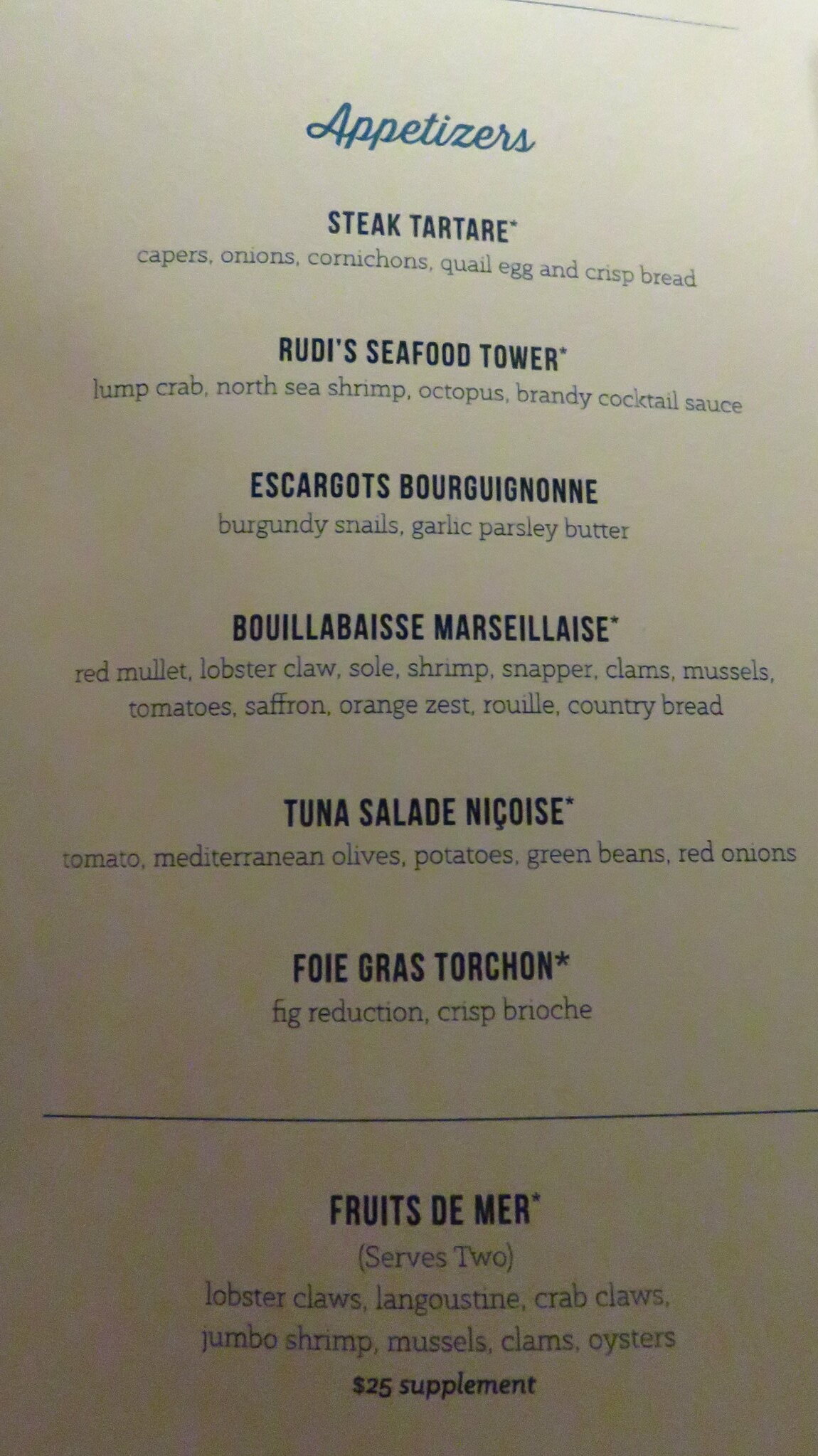This image depicts a sophisticated restaurant menu with a clean white background. At the top, in elegant blue cursive, it reads "Appetizers." The menu lists a series of appetizers, each in bold black text followed by detailed descriptions in lighter print. The appetizers include:

- **Steak Tartare**: Capers, cornichons, quail egg, and crisp bread.
- **Rudy's Seafood Tower**: Lump crab, North Sea shrimp, octopus, and brandy cocktail sauce.
- **Escargot Bourguignon**: Burgundy snails, garlic, parsley, and butter.
- **Bouillabaisse Marseillais**: Red mullet, lobster claw, sole, shrimp, snapper, clams, mussels, tomatoes, saffron, orange zest, and rural country bread.
- **Tuna Salmon Niçoise**: Tomato, Mediterranean olives, potatoes, green beans, and red onions.
- **Foie Gras Torchon**: Fig reduction and crisp brioche.
- **Fruits de Mer**: Serves two and includes lobster claws, clam crab claws, jumbo shrimp, mussels, clams, oysters, with a $25 supplement.

This concise yet rich description emphasizes the gourmet nature of the offerings, implying a high-end dining experience.